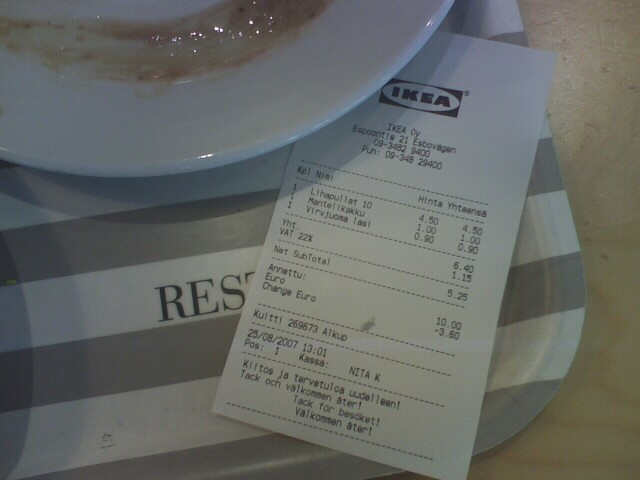The image depicts a dimly lit scene with an off-white counter in the foreground. In the upper left corner of the photo, there is a white plate that appears to be dirty, smeared with a brown sauce. Below the plate, a gray and white tray with horizontal stripes is visible, holding an Ikea receipt. The receipt is primarily white with black text. The recognizable Ikea logo is situated at the top, followed by text that appears challenging to read. One can make out some of the prices listed: $51.90, $5.40, and $1.15, likely in dollars and cents, though no dollar sign is explicitly shown. The text also includes a subtotal amounting to $5.25. To the left, the receipt mentions Euros and displays a non-final amount of "Euro $10" with a change calculated as a minus figure, possibly "-3.60". Several other lines of text remain unreadable due to the dim lighting and the language barrier.